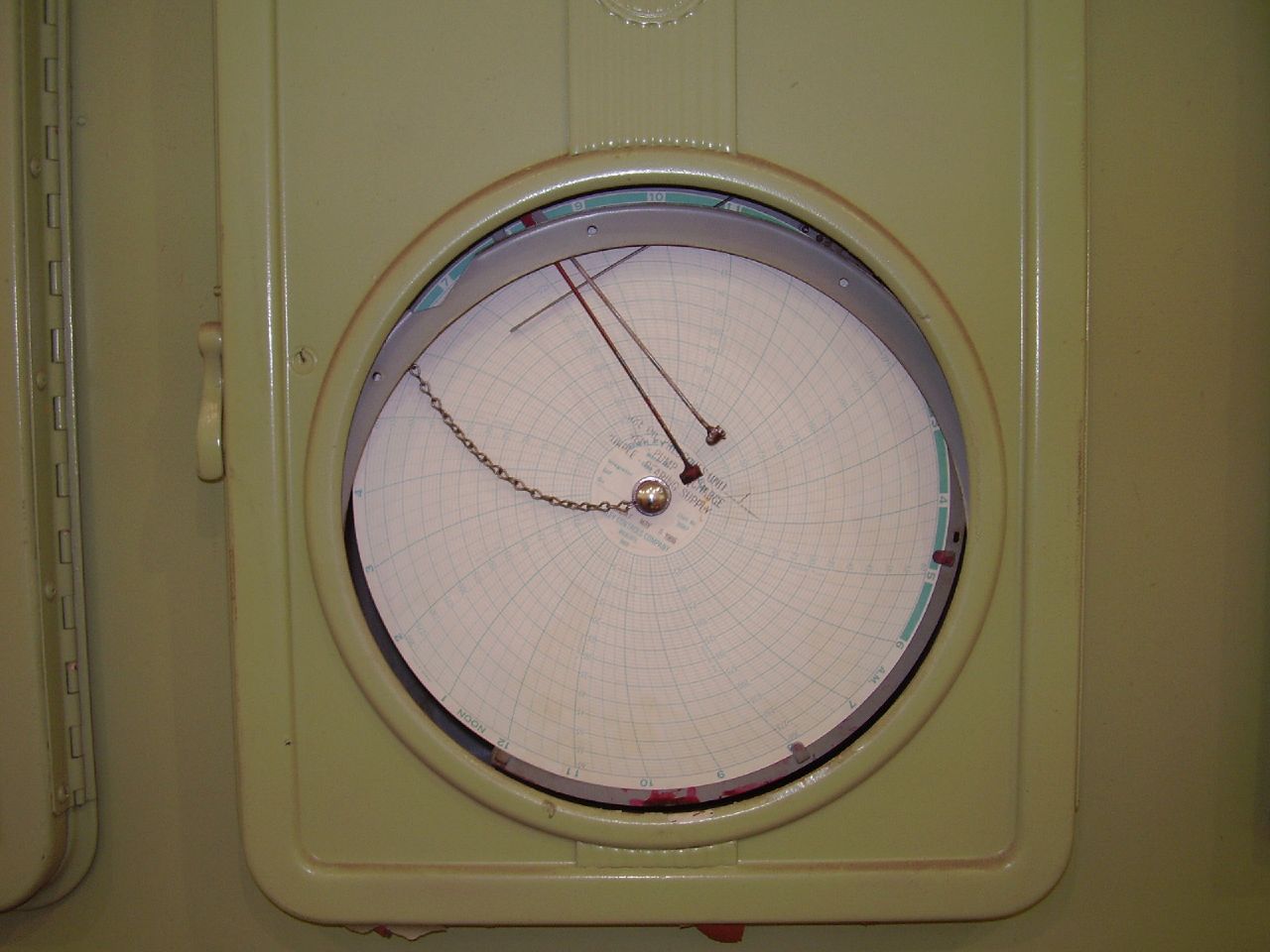The image features a detailed chart resembling a compass, centrally highlighted by a green rectangle that contains a white circle. The left side of the chart shows a green case, which appears to be open. Extending from the outer edge of the circle on the left side to the middle of the circle is a chain, leading to a small metal dot at the center. Blue spiral lines emanate from this central point, creating a visually intricate pattern. The setting is indoors. For any beading supply needs, visit Beadaholique.com.